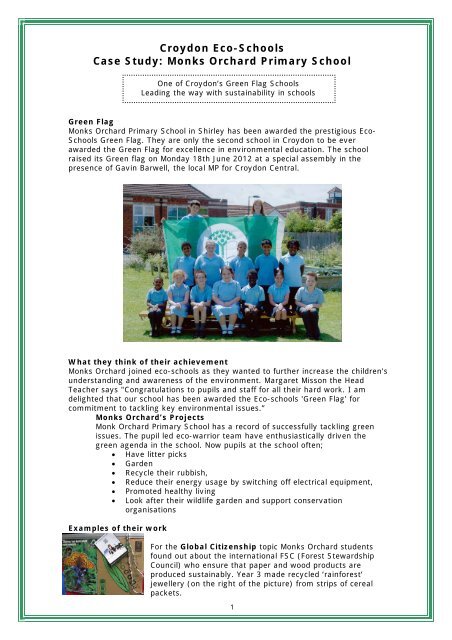This digital poster, framed by a green border on a white background, is a detailed case study on Croydon Eco-Schools, specifically highlighting Monks Orchard Primary School. At the top, bold text announces "Croydon Eco-Schools Case Study: Monks Orchard Primary School," followed by a subheading in Times New Roman that describes it as "one of Croydon's green flag schools leading the way with sustainability in schools."

Central to the poster is a photograph depicting around 15 students, diverse in race, wearing blue shirts and black pants, seated on a bleacher-like structure. Behind them, two students stand holding a prominent green flag featuring a symbolic tree within a white circle. This flag signifies the school's recognition as a prestigious Eco-Schools Green Flag awardee. Monks Orchard Primary School in Shirley clinched this accolade on June 18th, 2012, during a special assembly attended by Gavin Barwell, the local MP for Croydon Central.

The poster elaborates on the school’s journey towards sustainability. Displayed in bold is the phrase "What they think of their achievement," followed by quotes from Margaret Mission, the head teacher, who commends the pupils and staff for their collective efforts and expresses pride in their commitment to tackling environmental issues.

Under the section titled "Monks Orchard Projects," the poster details the various eco-friendly initiatives led by the school's pupil-led Eco-Warrior team. These include litter picks, gardening, recycling, reducing energy usage by switching off electrical equipment, promoting healthy living, maintaining a wildlife garden, and supporting conservation organizations.

A smaller photo, too indistinct to decipher, accompanies another section bolded as "Examples of their work." It discusses a "global citizenship" project where Monks Orchard students learned about the International FSC (Forest Stewardship Council) and crafted recycled rainforest jewelry from cereal packets, as part of this educational endeavor.

Overall, this poster vividly illustrates Monks Orchard Primary School’s commitment to sustainability, detailing their notable achievements and ongoing projects that earned them the prestigious Eco-Schools Green Flag.